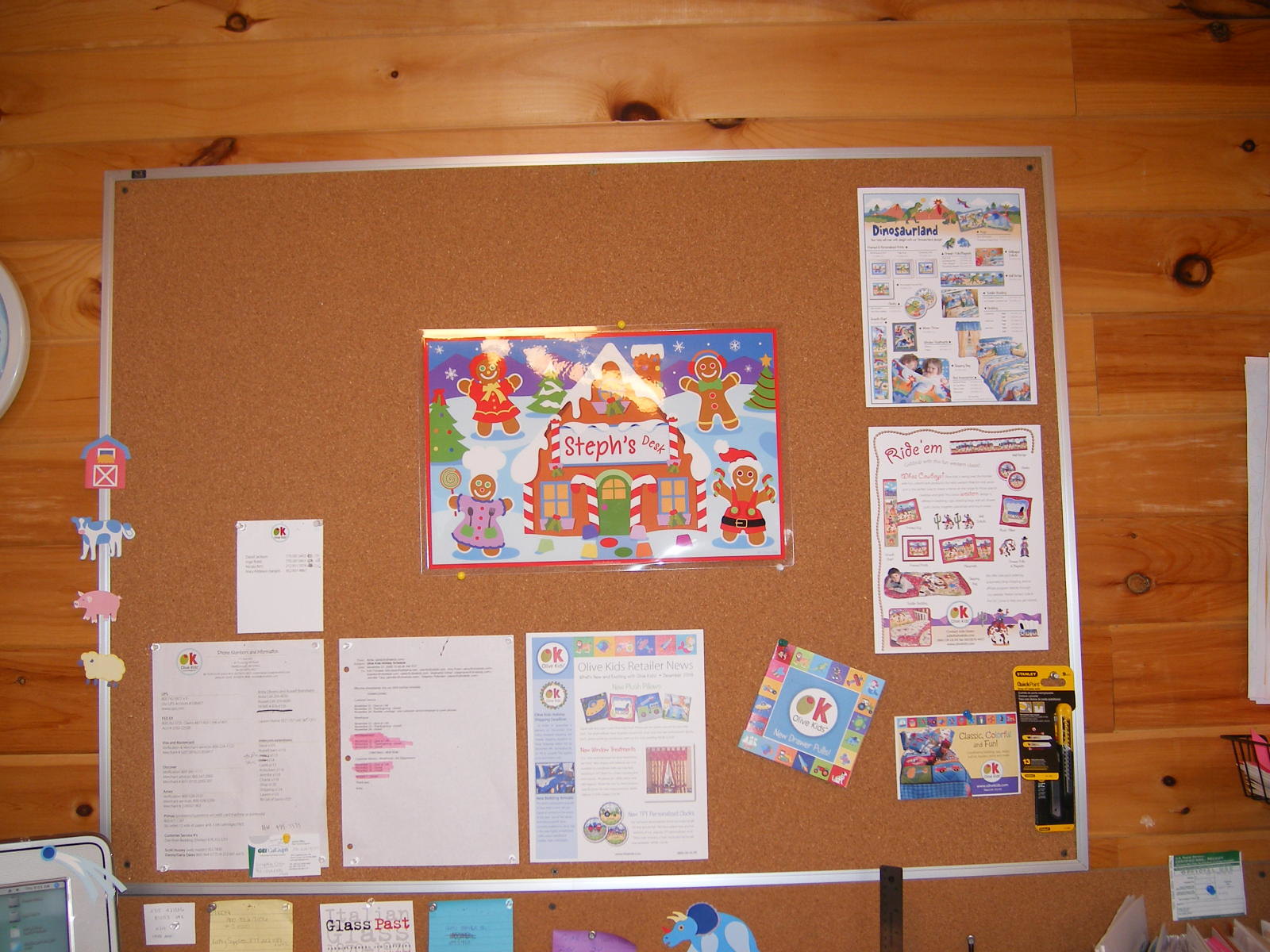The photograph features a large cork bulletin board with a thin metal border, prominently affixed to a wooden wall with horizontal, orange-toned planks adorned with numerous small knots. This bulletin board serves as a vibrant mosaic of various festive and informative postings. The centerpiece is a laminated picture of a gingerbread house, enveloped in a snowy nighttime scene, and adorned with four whimsical gingerbread figures dressed in varied Christmas costumes at each corner. The house bears a sign in red font reading "Steph's Desk". 

To the left of this central image, a series of cut-out farm animals—comprising a cow, pig, sheep, and a barn—accentuates the frame. Nearby hangs what appears to be a clock, partially visible. Additional noteworthy items on the board include a flyer for "Dinosaur Land" in the upper left corner, a promotional flyer labeled "Ride Um" below it, and another titled "Olive Kids Retail News". Scattered highlighters, colorful cards, office memos, and postcards add to the eclectic mix of postings. Beneath the main bulletin board resides another strip of cork festooned with further cards and cheerful, colorful animal stickers, enhancing the lively, community-centric feel of the scene.